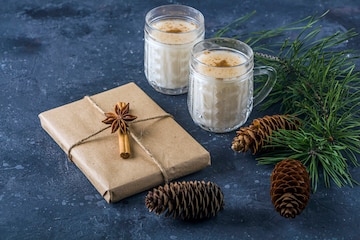In the image, a beautifully wrapped gift, possibly a book or photo frame, is the central focus. The gift is wrapped in rustic brown paper and adorned with twine, wrapped both longitudinally and latitudinally, creating a charming cross pattern. A cinnamon stick is attached as a decorative touch. Surrounding the gift, there are three pine cones and a small evergreen branch, contributing to a festive, natural feel. Flanking the scene are two milky white candles in glass holders, enhancing the cozy ambiance. Completing the holiday setting, two creamy beverages, which appear to be eggnog sprinkled with nutmeg, are placed nearby. The entire arrangement is set against a blue surface, evoking a serene and inviting atmosphere perfect for a holiday gathering.